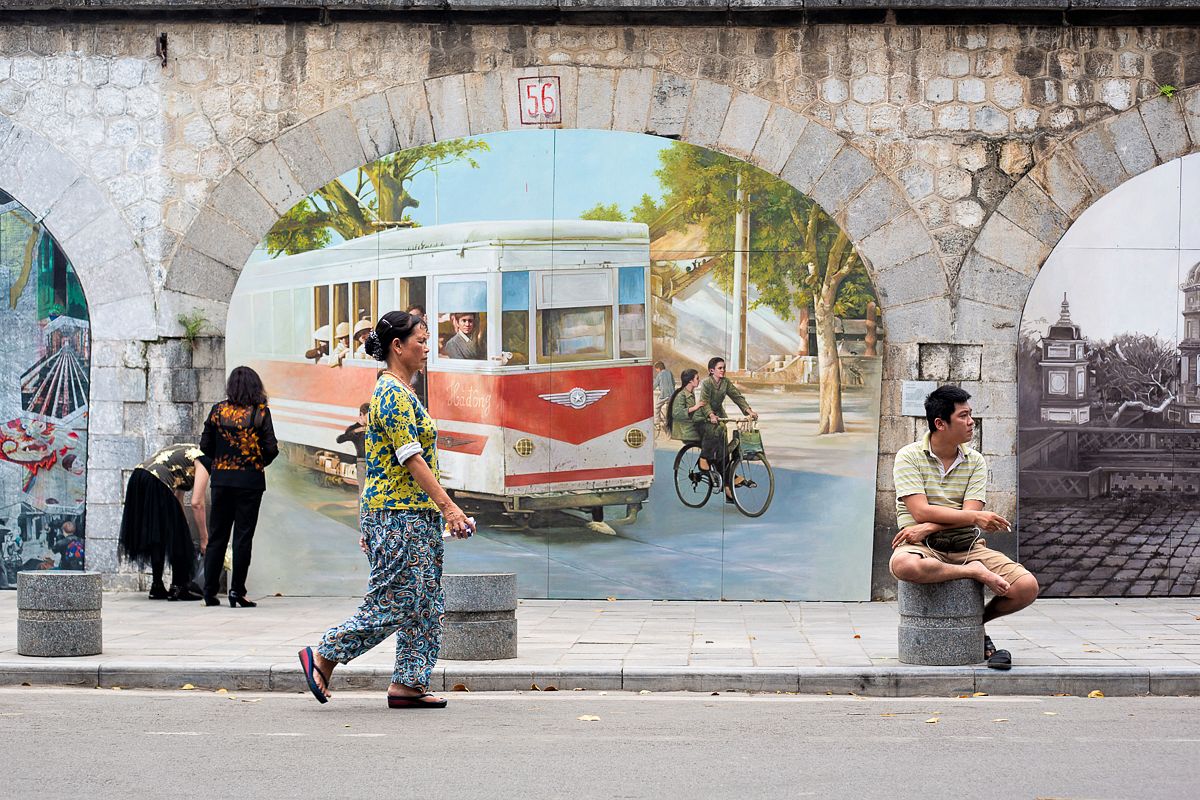This detailed color photograph captures a bustling street scene outside with intricate urban elements. The foreground features an asphalt road running horizontally, where a woman clad in a vibrant floral blue and yellow top, along with elaborately patterned pants and sandals, strides from left to right. Parallel to the road, a slightly raised curb delineates a stone tile sidewalk populated by several figures. On the left side of the image, two women dressed in black stand; one in black slacks, the other in a black skirt, with the latter bent over rummaging through her bag. To the right, a man in tan shorts and a lime green striped shirt with a cigarette in his right hand sits confidently on a short pillar, his right leg propped atop it while his left balances on the ground.

Dominating the background is an arched stone brick wall bearing the number 56 atop its central arch. This segment of the wall showcases a large, detailed mural of a city tram—white or cream with striking red stripes—capturing the essence of urban transit with visible overhead wires. Within the tram, passengers can be seen, notably a person in the front window and several individuals further back, distinguished by their tan hats. The mural also includes scenes of the city, possibly featuring people riding bicycles, adding to the dynamic composition of this lively street snapshot. The stone arches flanking the mural reveal sections of the wall's original grey and brown brickwork, intensifying the rich textures and stories embedded in this urban tableau.